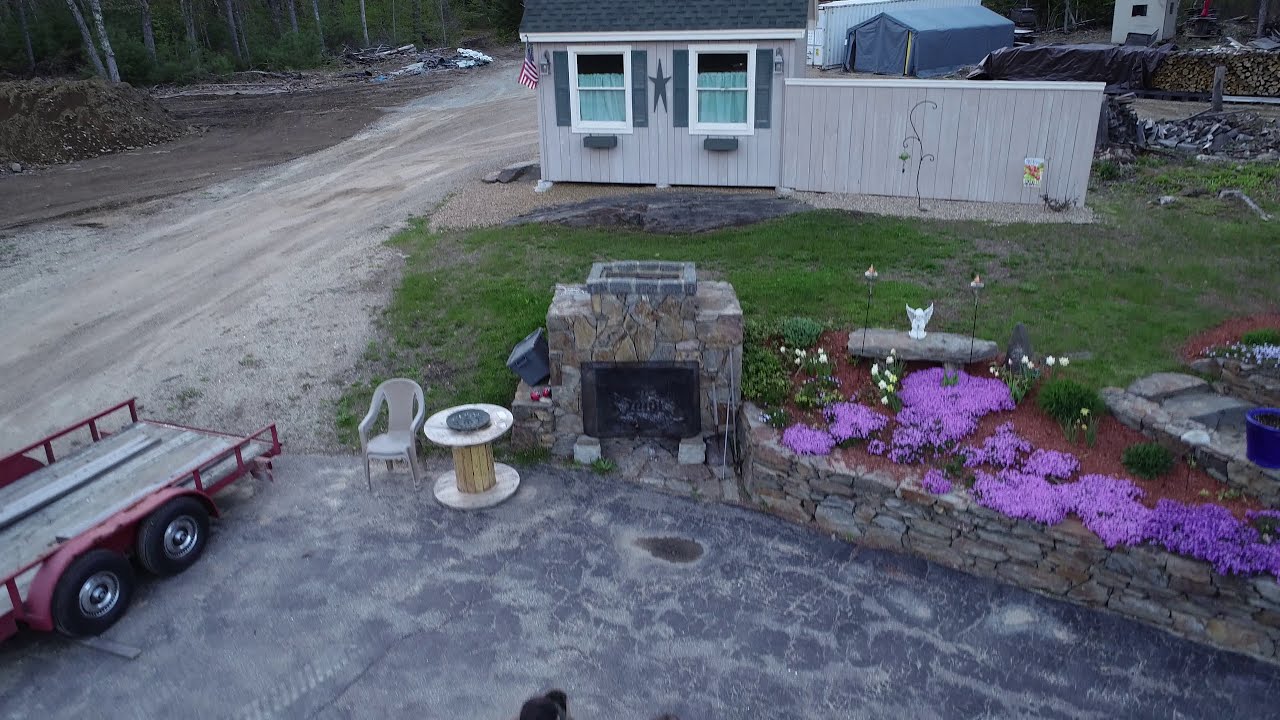This image depicts an outdoor setting that appears to be someone's backyard during the daytime. Central to the image is an outdoor fireplace, with its position closest to the middle of the photo. In the bottom left corner, the back of a large trailer, designed for carrying a car and fitted with two axles, is visible. Nearby, a plastic patio chair sits next to a repurposed wooden cable spool used as a table. Alongside these objects, a dirt road stretches into the distance, flanked by trees.

In the background, there is a shed, and within the space, a small garden area features red wood chips with a variety of flowers, including purple and violet ones, adding a splash of color. The garden is further embellished with a statue of an angel perched atop a large stone. The house, situated towards the rear and center of the image, is gray with wooden siding, displays an American flag on the left side, two windows, and a dark blue star between them. The blinds on the windows are light blue, and a brick oven or similar structure is stationed in front of the house.

The overall color palette includes tan, red, black, pink, purple, green, and gray, contributing to the cozy and eclectic feel of the backyard. True to its setting, there is no readable text within this image.